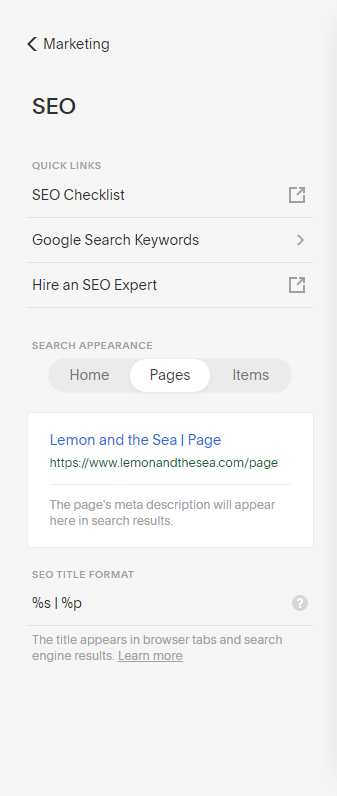In the image of a marketing website's interface, a section at the bottom of the page displays an area labeled "SEO" nestled within a "Quick Links" section. The "Quick Links" section appears in smaller gray text. Directly below this, in bold black text, is the "SEO Checklist," accompanied by an icon of a box with a diagonal arrow pointing upwards, indicating an external link. 

Next in the list is "Google Search Keywords," marked with a rightward-pointing arrow. Following this is the option "Hire an SEO Expert." 

Further down, there's a section titled "Search Appearance" with navigation options including "Home," "Pages," and "Items." The "Pages" button is highlighted in white, making it prominent compared to the other two gray, flush icons. 

Beneath the "Pages" button is a blue-highlighted label, "Lemon In The Sea," followed by a green URL: "www.lemoninthesea.com/page." Below this green URL, in gray text, is a placeholder for the meta description that reads, "The page's meta description will appear here in the search results."

Further down is another section labeled "SEO Title Format," which contains a string of mixed characters like percentages, S's, and question marks, culminating in a clickable icon to the right. Below this section, a note reads, "The title appears in browser tabs and search engine results. You can learn more."

The interface's entire background is light gray, except for the "Lemon In The Sea" box and the "Pages" button, which both feature a white background, making them stand out.